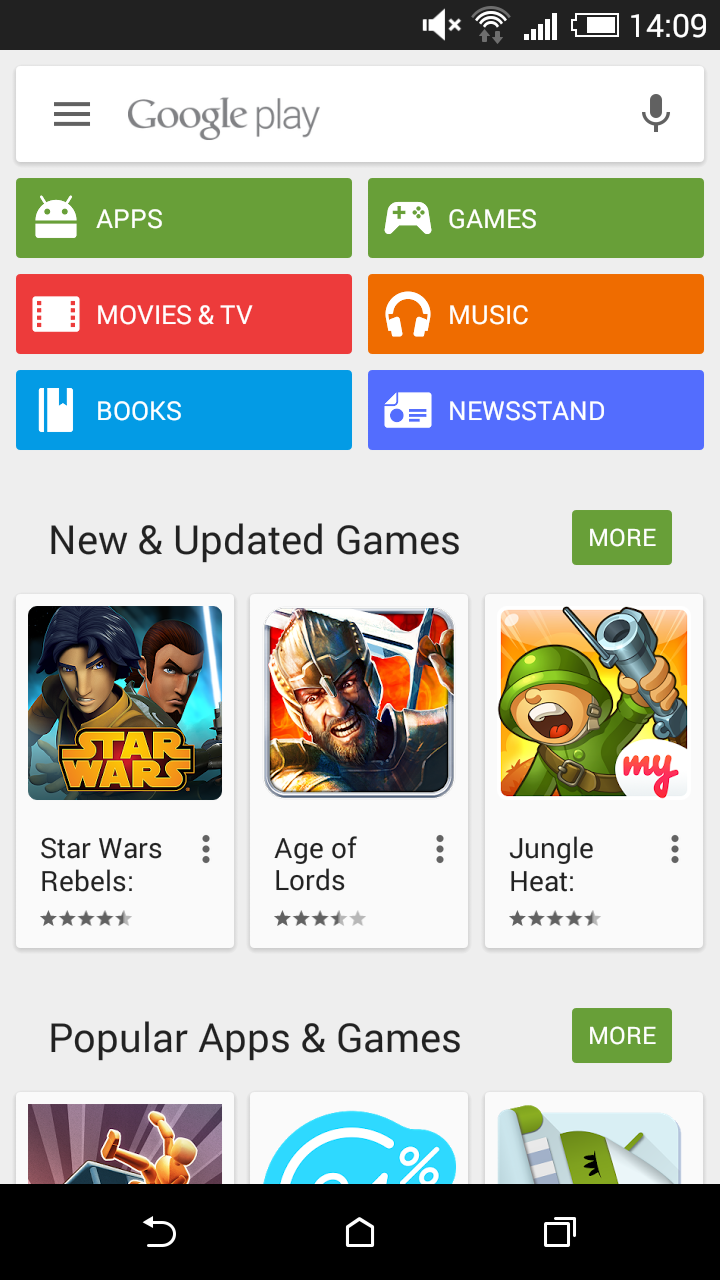In the top right corner of the image, there is an almost fully charged battery icon, and the time is displayed as 14:09. Below that, a prominent white bar labeled "Google Play" spans the width of the screen. On the left side of this bar are three horizontal lines, commonly representing a menu, while on the right side is an icon of a microphone.

Beneath the main bar, there are several subcategories listed: Apps, Movies & TV, Books, Games, Music, and Newsstand. Following these subcategories, a section titled "New and Updated Games" features with an option to click on a green square labeled "More."

Under this section, there are images and details of various games. For instance, one image shows two characters wielding lightsabers with the title "Star Wars Rebels," rated 4.5 out of 5 stars. Another image features a knight holding a sword under the title "Age of Lords," rated 3.5 out of 5 stars. Additionally, an image showing a character in an army hat and uniform under the title "Jungle Heat" is rated 4.5 out of 5 stars.

Further down, another section titled "Popular Apps and Games" appears with an option to click on a green square labeled "More," similar to the one above.